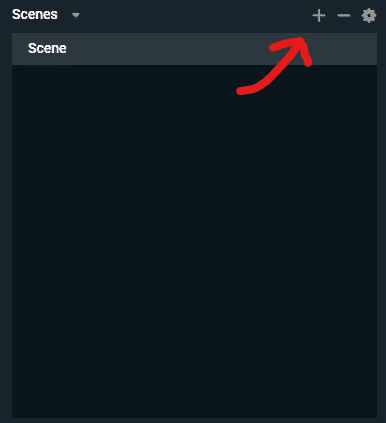The image is a screenshot predominantly characterized by dark tones. It features a nearly square black rectangle as the main background. Encasing this black rectangle is a dark gray border.

Near the top of the image, just slightly down from the edge, there is a dark gray bar stretching horizontally across the screen. In the upper left-hand corner of this bar, the word "Scenes" is prominently displayed in white text, accompanied by a clickable downward-pointing arrow next to it. Directly below this, within the same dark gray bar, the word "Scene" also appears.

In the upper right-hand corner of the dark gray bar, there are three icons lined up: a plus sign, a minus sign, and a gear icon, all in white.

A hand-drawn dark red arrow, added digitally, points directly to the plus sign in the upper right-hand corner, drawing attention to this particular icon. The minimalistic design and focused details create a clear, yet visually subdued, screenshot.